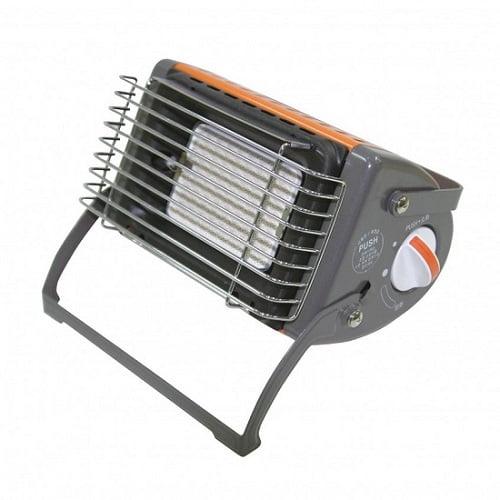The image showcases a compact, gray, and metallic floodlight or possibly a portable heat lamp, positioned against a white background. The device features an orange top and a prominent gray handle affixed with screws, allowing for easy portability and adjustment. It has a distinctive wire screen or metal grate covering a square, headlight-like section, which might also serve as a protective casing for a heating or lighting element. Below the metal grate, there is a white rectangular area that could be the light or heat source. This unit is equipped with a white knob featuring an orange line, located on the side, which appears to adjust settings, with the word "PUSH" labeled nearby. Additionally, the device has two different handles designed for versatile positioning, enhancing its practicality in various field applications. The overall size of the unit seems relatively small, making it highly portable.